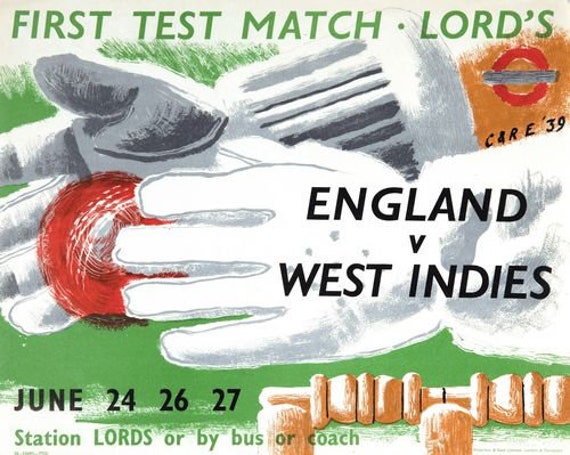The image is an illustrated advertising poster for the first test match of a cricket series between England and the West Indies. Central to the image is a pair of hands wearing white gloves with some gray in the palms, holding a small red cricket ball. Prominently displayed at the top is green text that reads, "First Test Match • Lord's," with "Lord's" containing an apostrophe S. Below this is a logo featuring a red circle with a gray horizontal bar through it, alongside the text "CNRE39" in a handwriting font. The white gloves also display the text "England vs. West Indies" in black. Towards the bottom of the poster, the dates "June 24, 26, 27" are written in black against a green background. Further down, "Station Lord's, or by bus or coach" is noted in green text on a white background. In the lower left-hand side of the image, there's a series of brown shapes lined up in a row, and on the right side, there’s a depiction of the cricket stumps with the bails balanced on top, indicating it is indeed a cricket match.